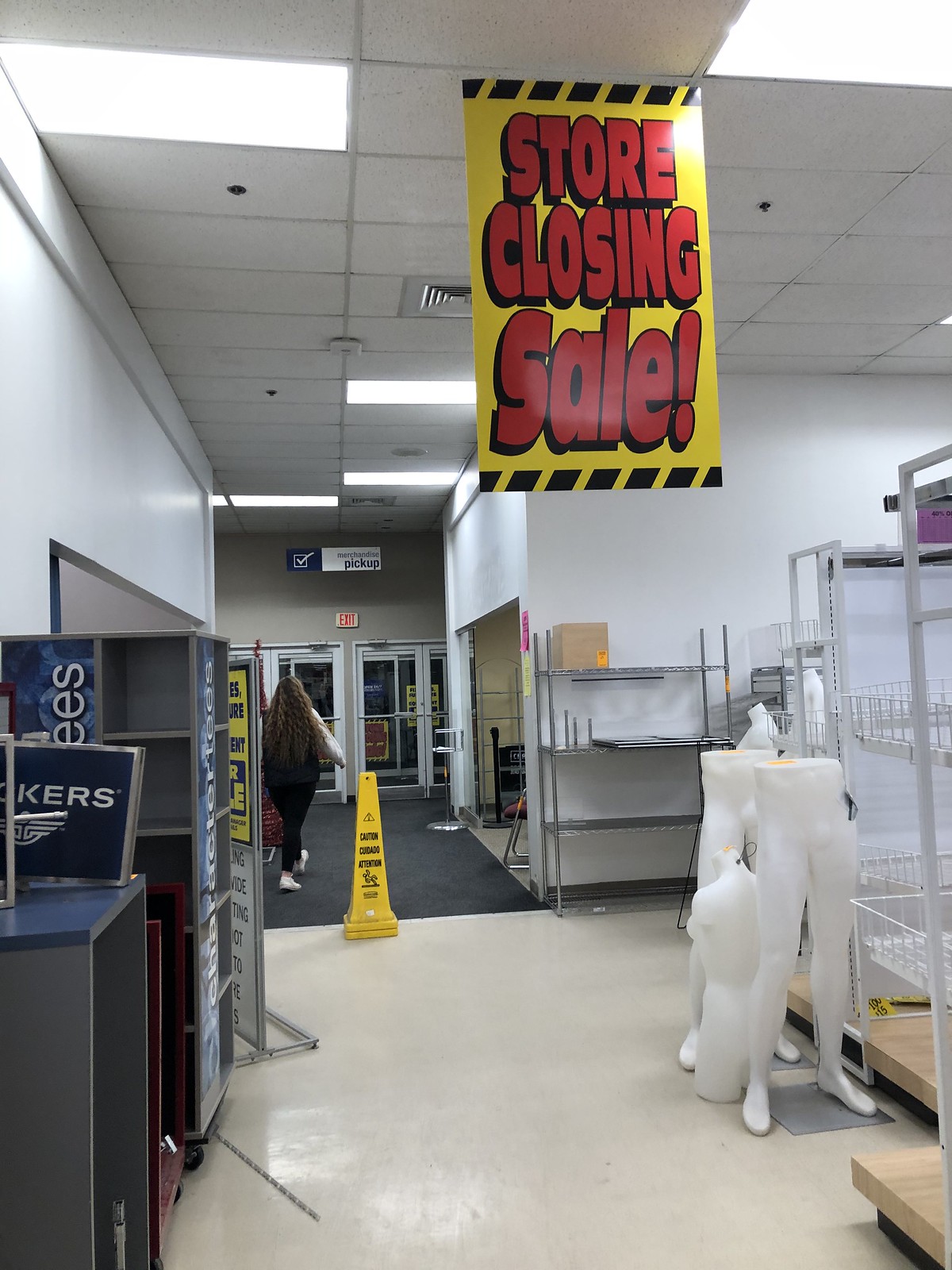The photograph, taken inside a nearly empty store that has gone out of business, captures an atmosphere of desolation and abandonment. Dominating the scene is a bright, yellow sign with bold red lettering that reads "Store Closing Sale," hanging prominently from the ceiling. The store's off-white tile floor transitions to black carpet toward the back. A vivid yellow caution wet floor cone stands conspicuously on the white tile. Silver metal shelves and racks, stripped of merchandise, line the space, with signs of brands like Dockers and a partially visible Skechers sign ("-K-E-R-S") hinting at what once was on display. Disassembled mannequins lie scattered: two lower torsos upright and one upper torso forlornly on the ground. The store's ceiling features white panels, square lights, a white vent, and fire sprinklers. To the left, gray stands and some blue signs add to the dreary tableau, while brown counters and silver stands can be seen on the right. In the background, the storefront's silver-colored doors are marked by a red exit sign above, accompanied by a white and blue "Pickup" sign. A woman, clad in a white shirt, black vest, black pants, and white shoes, is caught mid-stride on the black carpet, making her way out of the empty shell of the former bustling retail space.